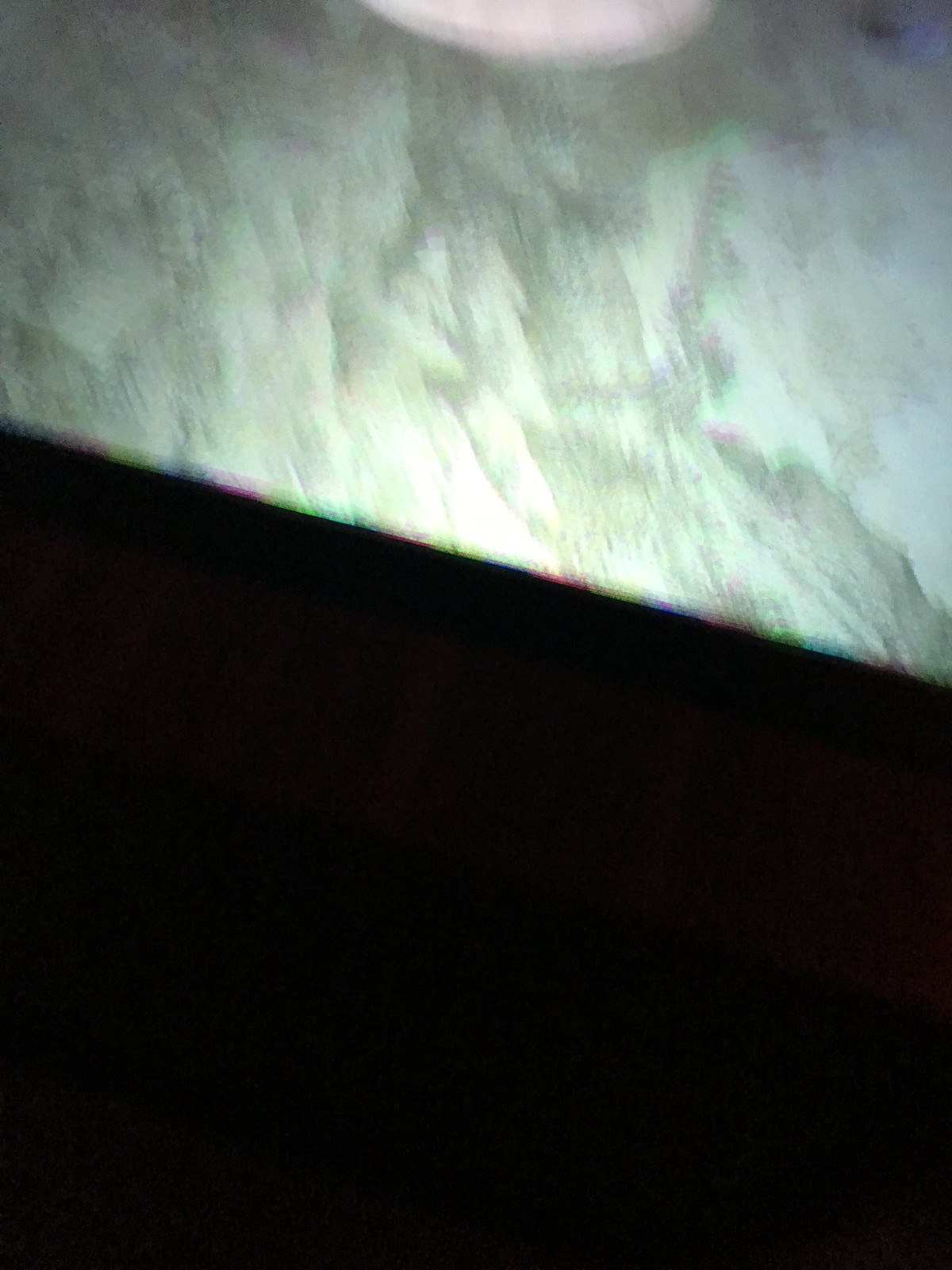This highly blurry and out-of-focus photograph displays a vague, up-close scene with a stark contrast between two distinct halves bisected diagonally. The bottom half of the image is pitch black, seemingly indistinguishable, likely due to an absence of light. The top half showcases a textured, vaguely circular object with a mixture of bluish-green, light brown, and splotchy patterns. This object, though hard to identify, might suggest a surface such as a mattress or possibly the sill of a window with an exterior element, like light or snow, trying to penetrate through. The top edge features a thin strip of rainbow colors, adding an elusive hint of light or refraction. The limited lighting and the extreme close-up nature of the shot render the image’s content ambiguous, adding a mysterious quality to the scene.